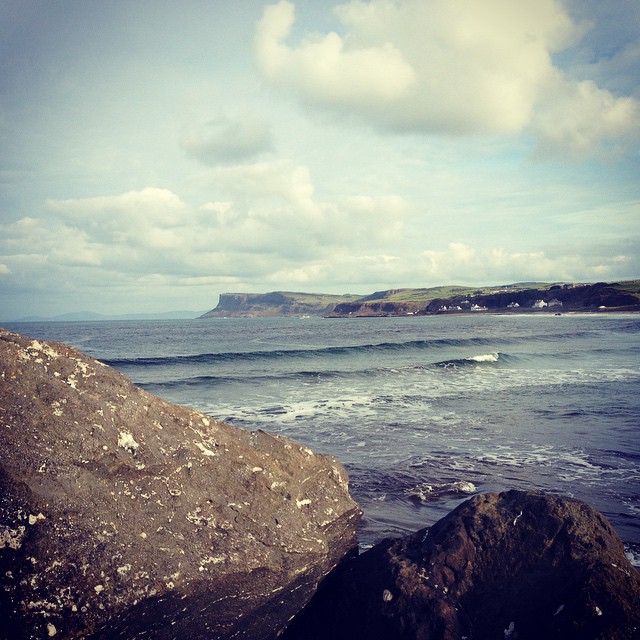An outdoor photograph captures a serene seaside scene at daytime. In the foreground, two prominent rocks dominate the lower part of the image; the larger rock on the left is a lighter gray speckled with white, while the smaller rock on the right has a dark gray and brown hue. Sunlight gently illuminates these rocks, adding a warm glow. These rocks give way to an expansive body of ocean water with gentle waves rolling towards a sandy shoreline. Just beyond the shore lies a green, flat landmass that appears sharply elevated from the sea, bordered by a distant mountain range on the left. Scattered throughout the blue sky are fluffy white and gray clouds. In the far distance, white houses can be seen perched by the sea, adding a touch of human presence to the natural scenery.